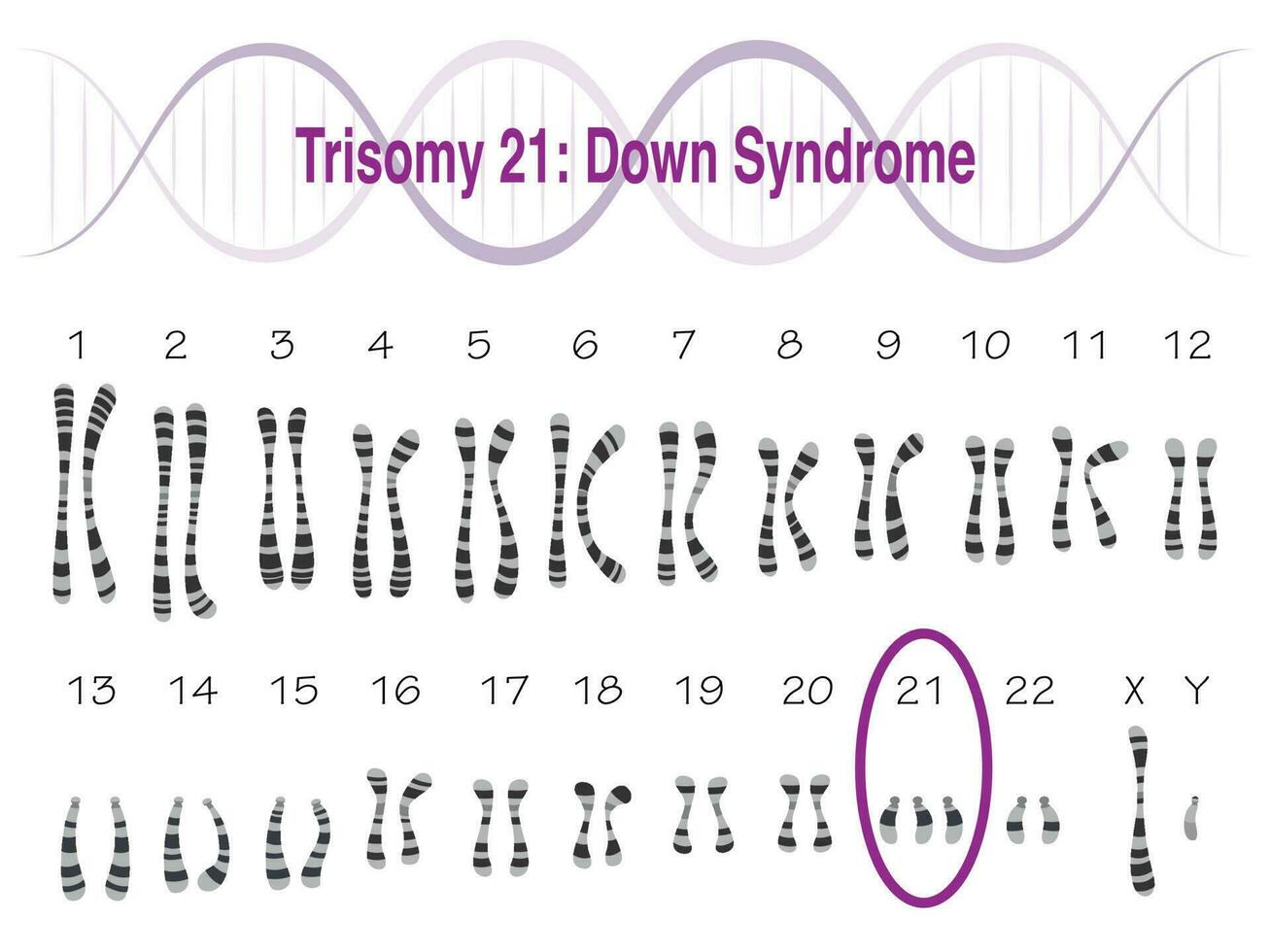The image depicts a detailed illustration of chromosomes associated with Down syndrome, specifically Trisomy 21. At the top, there is a header in purple text that reads "Trisomy 21: Down syndrome" with a background of wave-like DNA sequences rendered in gradient shades of purple, gray, and white. Below this header, the chromosomes are organized in three rows, numbered 1 through 22. The chromosomes appear as gray and black striped shapes resembling gummy worms. The key feature is the 21st chromosome, circled in purple, which highlights its significance in Down syndrome. The chromosomes are shorter compared to the others, emphasizing the genetic anomaly. The comprehensive layout visually explains the genetic differences in individuals with Down syndrome.